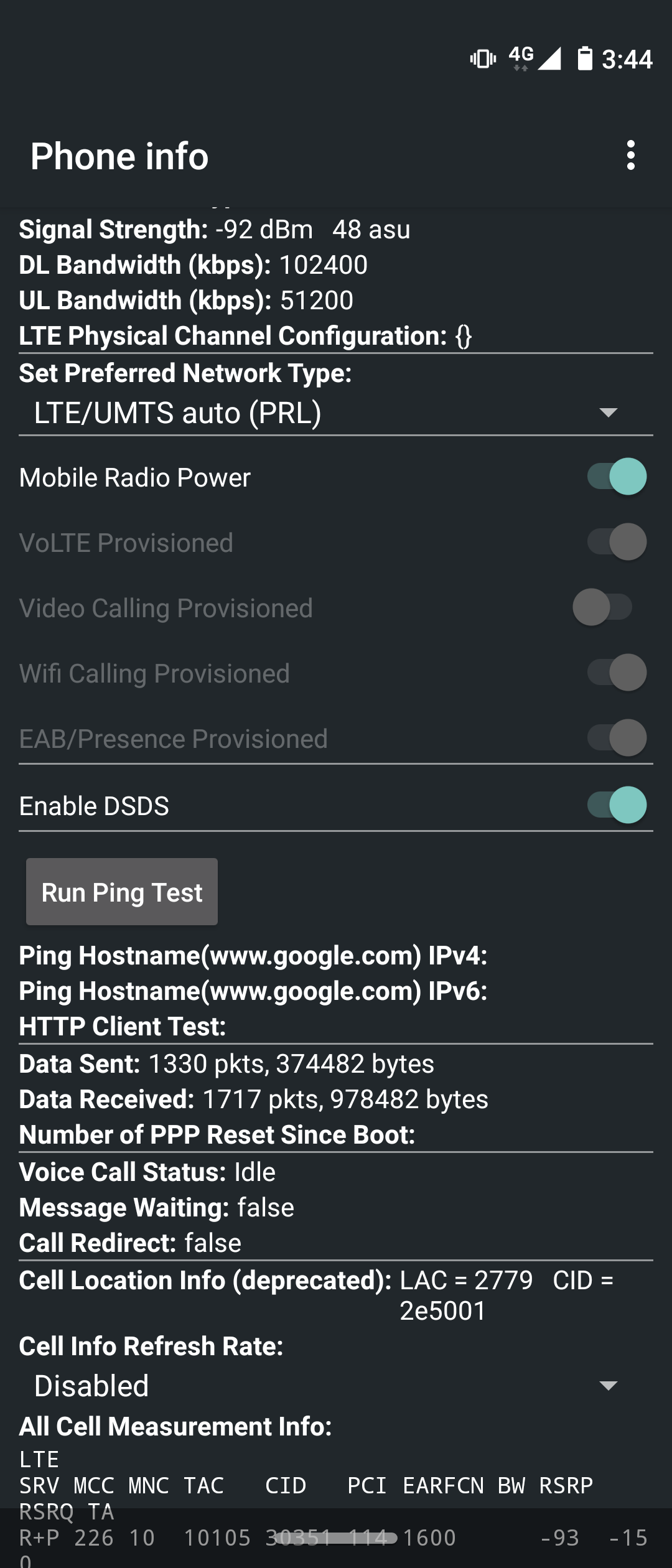The image depicts a detailed debugging screen of a mobile phone's network settings. The background is black, while the text and interface elements are primarily green, gray, and white. At the top, the current time is displayed as "3:44". Below this, the phone's signal strength is shown as "-92 dBm", accompanied by a capital "B" with "48 ASU". 

The DL (download) bandwidth is listed as "102400 KBPS" and the UL (upload) bandwidth as "51200 KBPS", both enclosed in parentheses. The network type is specified as "LTE" with physical channel configuration details provided, but the specifics are contained within two brackets. 

Further down, there is an option to "Set Preferred Network Type" which is set to "LTE/UMTS auto (PRL)". The "Mobile Radio Power" option is also present, with a blue toggle bar indicating it is turned on.

In white text on gray background, several toggle options are displayed:
- "VOLTE provision" toggle bar is on.
- "Video calling provision" toggle bar is off.
- "Wi-Fi calling provision" toggle bar is on.
- "EAB/Presence provision" toggle bar is on.

Additionally, the "Enabled DSDS" function is shown with a white toggle bar, which is also on. At the bottom of the screen, there is an option labeled "Run Ping Test" displayed in white text on a gray rectangle.